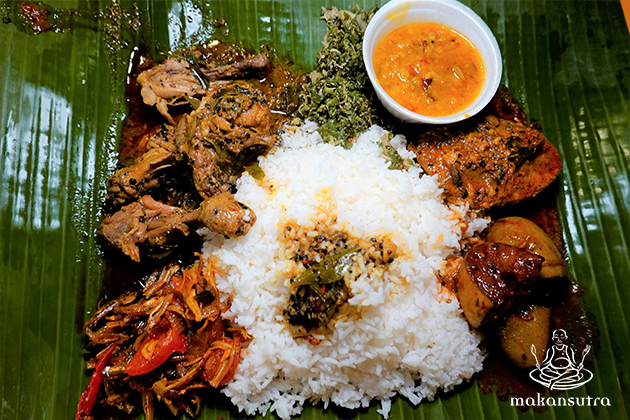The image showcases a traditional meal beautifully arranged on a large green leaf, resembling bamboo leaves, used as a rustic plate. In the center of the leaf lies a generous mound of white rice, adorned with various seasonings and a vibrant salsa that appears to have a teriyaki hue. Surrounding the rice, there is an assortment of colorful, finely chopped vegetables, reminiscent of the texture of canned spinach, adding to the intricate detailing of the dish.

To the left, tender pieces of chicken, likely seasoned with teriyaki sauce, are mingled with chunks of tomatoes. Adjacent to them, a cluster of well-seasoned mushrooms complements the savory profile of the meal. Positioned beside the main arrangement is a small, clear plastic container holding a brown-orange liquid, possibly a mango salsa, adding a sweet and tangy element to the dish.

At the bottom right corner of the setup, an emblem of a person sitting cross-legged with a fork and spoon in each hand, accompanied by the text "Makkan Sutra," adds a cultural touch to the presentation. The detailed seasoning spread across the dish enhances its visual appeal, making it look absolutely delectable.